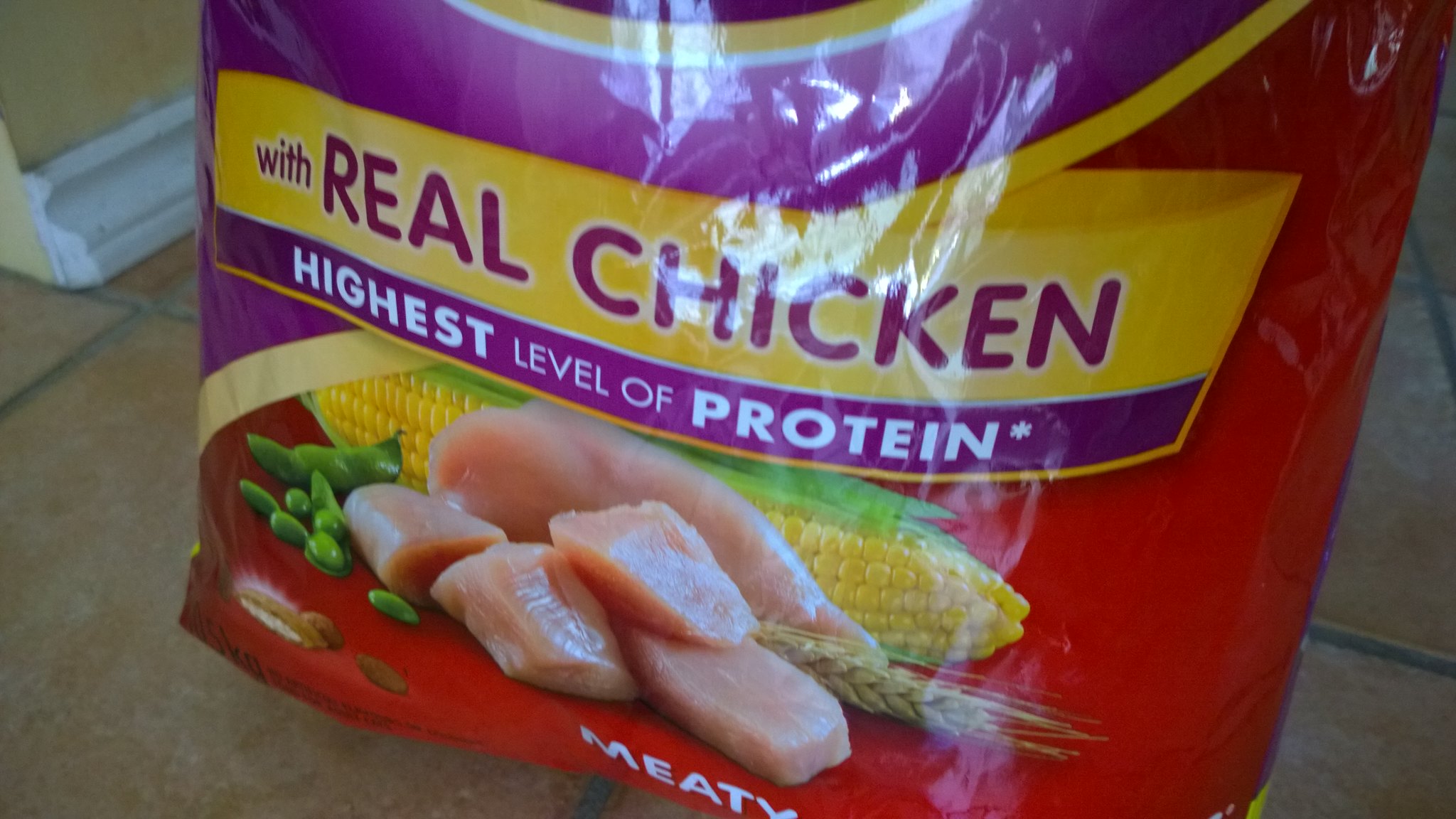A detailed photograph showcases a large, shiny package of pet food, visibly placed on a beige tile kitchen floor. The reflective packaging, predominantly adorned in red, purple, and yellow hues, prominently features text stating, "With Real Chicken, Highest Level of Protein." Accompanying this text is an appetizing image of ingredients, including corn, peas, chicken, and wheat, with the word "Meaty" displayed beneath them. The top left corner of the image reveals a fragment of a yellow painted wall and a section of white baseboard, suggesting that the setting is likely within a domestic kitchen. There are no people present in the picture.